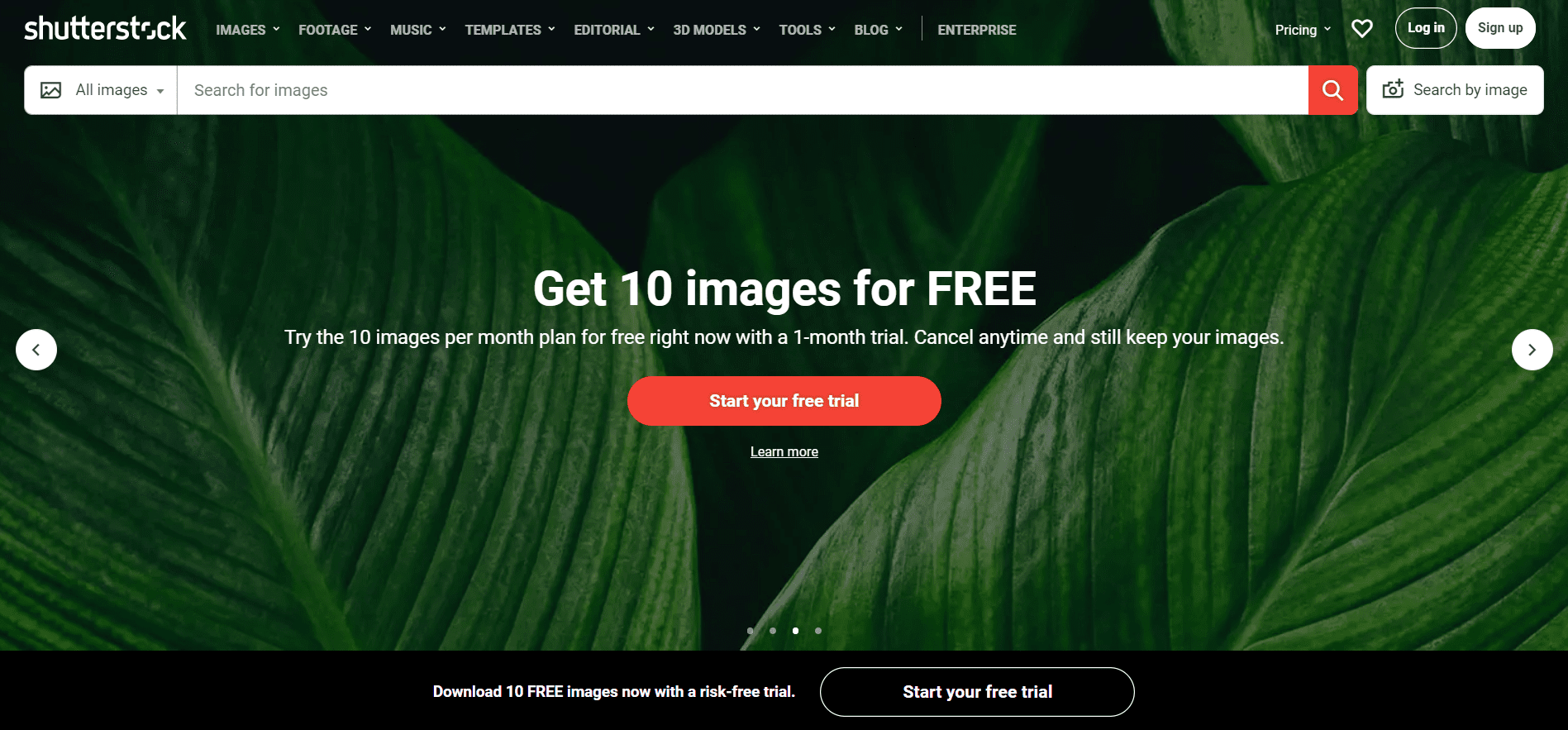The webpage in the image features an interface offering various stock resources, including images, categories, footage, templates, editorial content, 3D models, and tools. At the top, there are links to a blog, enterprise solutions, pricing details, login, and sign-up options. The center prominently displays a search field labeled "search for images," with an adjacent button labeled "all images."

Below the search field, the webpage promotes a free trial offer: "Try the 10 images per month plan for free right now with a one-month trial. Cancel anytime and still keep your images." Additional buttons encourage starting the free trial and downloading 10 free images without risk.

The color scheme of the webpage incorporates green, red, black, and white elements, creating a visually engaging and user-friendly experience.